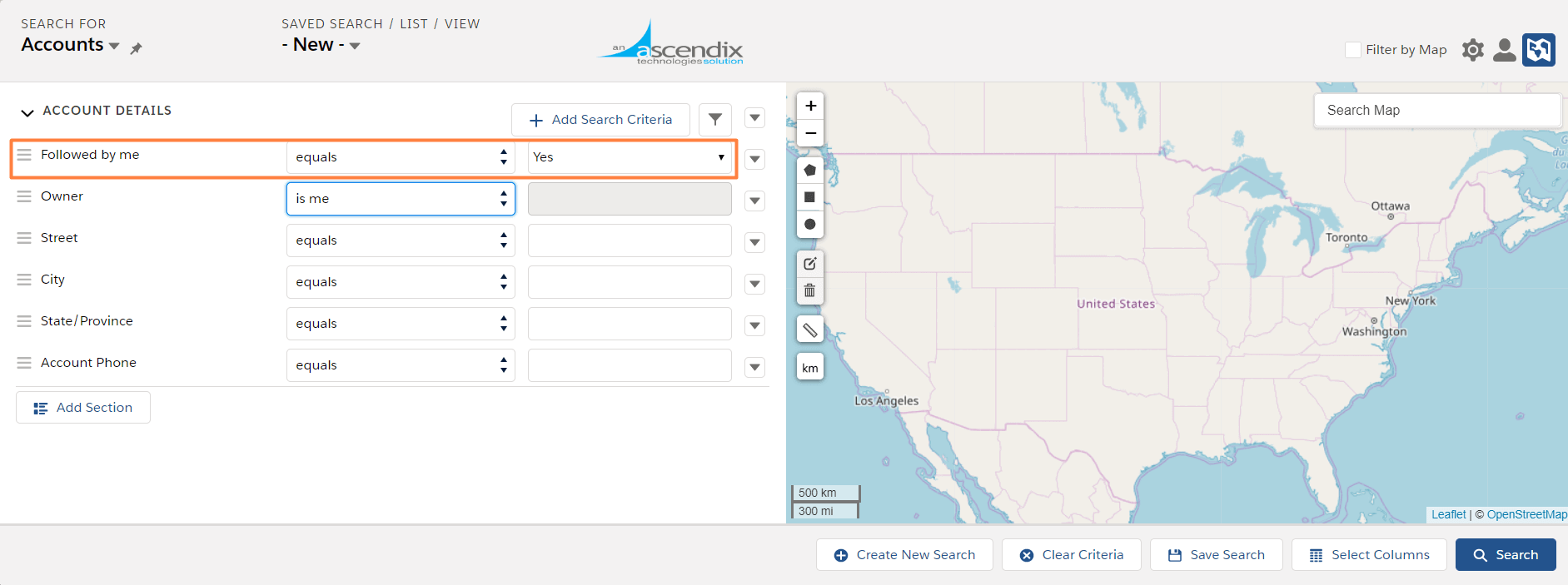**Detailed Caption for the Ascendix App Image:**

The image depicts a screenshot of an application interface called Ascendix, designed to function across a wide screen with a resolution approximately double that of a standard tablet, side-by-side. Despite its somewhat low resolution, the text remains legible. The layout of the app features several distinct sections:

- **Top Banner:** This begins with a dropdown menu labeled "Search for accounts." Next to this are buttons for "Save search," "List view," and "New," which also has a dropdown menu. In the center of this banner is the Ascendix logo. To the right, text reads "Filter by map" followed by a checkbox, a settings gear icon, a simplified user icon, and finally, a blue map icon featuring white map line drawings.

- **Left Panel:** This gray section is a square panel whose contents are not described in detail.

- **Middle Section:** This area has a white background and contains the primary content of the app. The section titled "Account Details" displays six columns: "Followed by Me," "Owner," "Street," "City," "State/Province," and "Account Phone." These columns are used to add and refine search criteria, providing a clear template for data organization.

- **Right Panel:** Displaying a map of the United States with surrounding areas of Mexico and Canada in gray, and bodies of water depicted in light blue. 

Within the "Account Details" section, a specific feature is highlighted for demonstration purposes: the "Followed by Me" column features a menu labeled "Equals" with two arrows, and the option "Yes," which is encased in a red box indicating it’s an example or point of focus.

This image likely serves as a demonstration tool to showcase the app's functionalities and user interface elements.